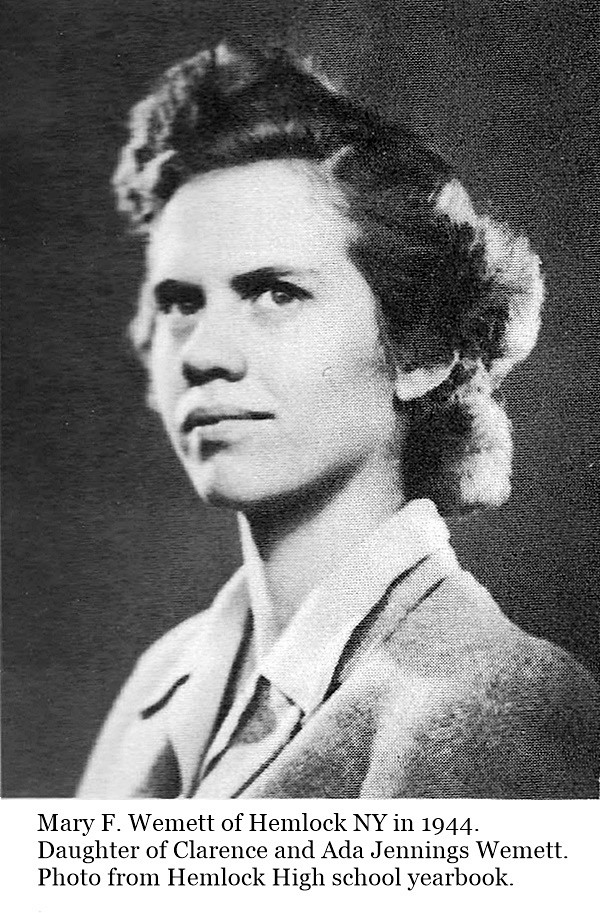This is a black and white headshot of Mary F. Wemmett of Hemlock, New York, taken in 1944 for the Hemlock High School yearbook. The text beneath the photo indicates that she is the daughter of Clarence and Ada Jennings Wemmett. Mary is depicted with short, thick brunette hair styled in a quintessentially 1940s fashion, parted on the side, curled, and puffed up on top. She appears intensely serious, with dark eyes and a straight-line mouth adding to her determined expression. She is dressed in a collared blouse topped with a buttoned woolen jacket that resembles tweed. Despite being a high school yearbook photo, Mary has a mature appearance, seeming older than her high school years. The background of the photo is black, which emphasizes her focused and poised demeanor.